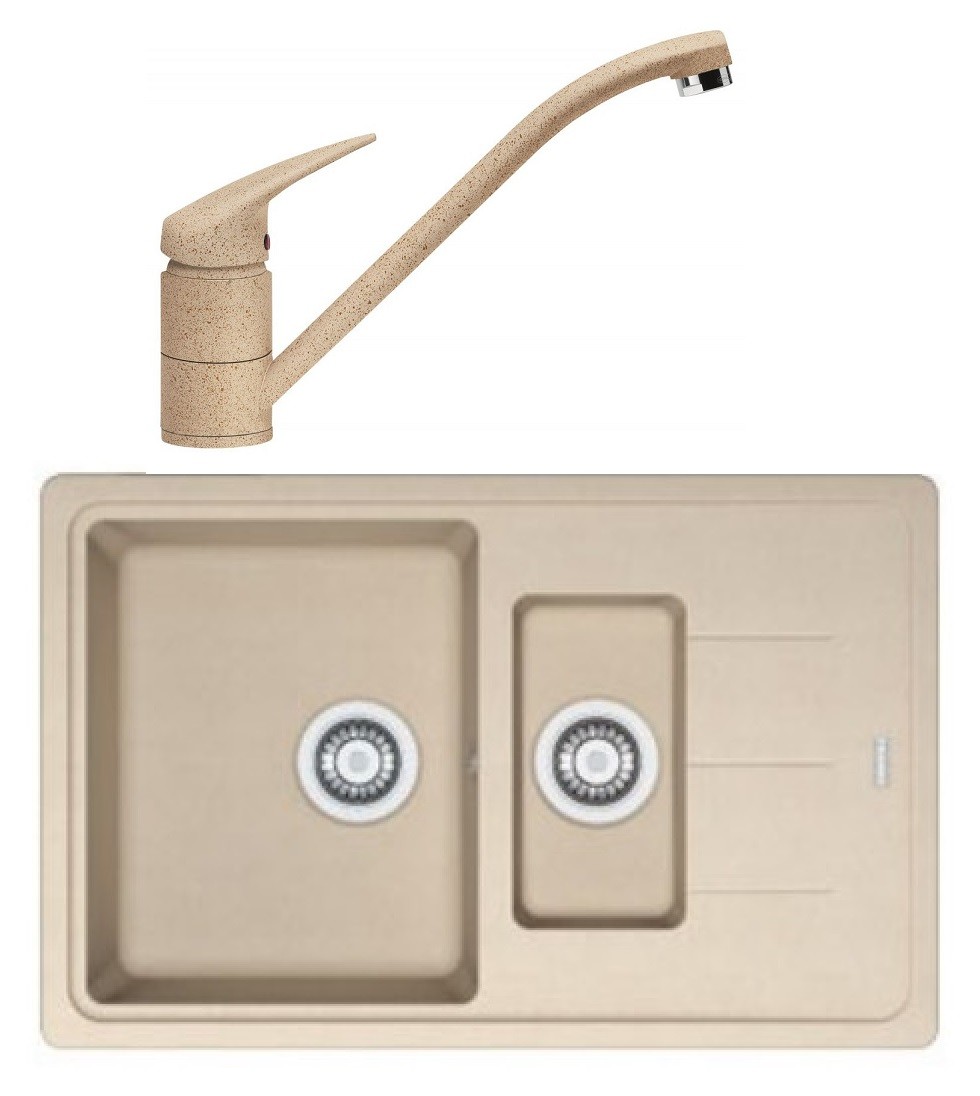The image is a composite photograph illustrating a matching kitchen sink and faucet set. The peach-colored sink features a large basin with a chrome drain plug on the left side and a smaller, rectangular basin with a chrome drain plug on the right, alongside a flat preparation area with shallow grooves that likely help in draining water. The faucet is shown separately in a profile view above the sink from an aerial perspective. It is similarly peach-colored, adorned with red speckles, and has a silver-colored spout. This cohesive design suggests that the sink and faucet are part of a coordinated set, with the faucet's aesthetic closely matching that of the sink.